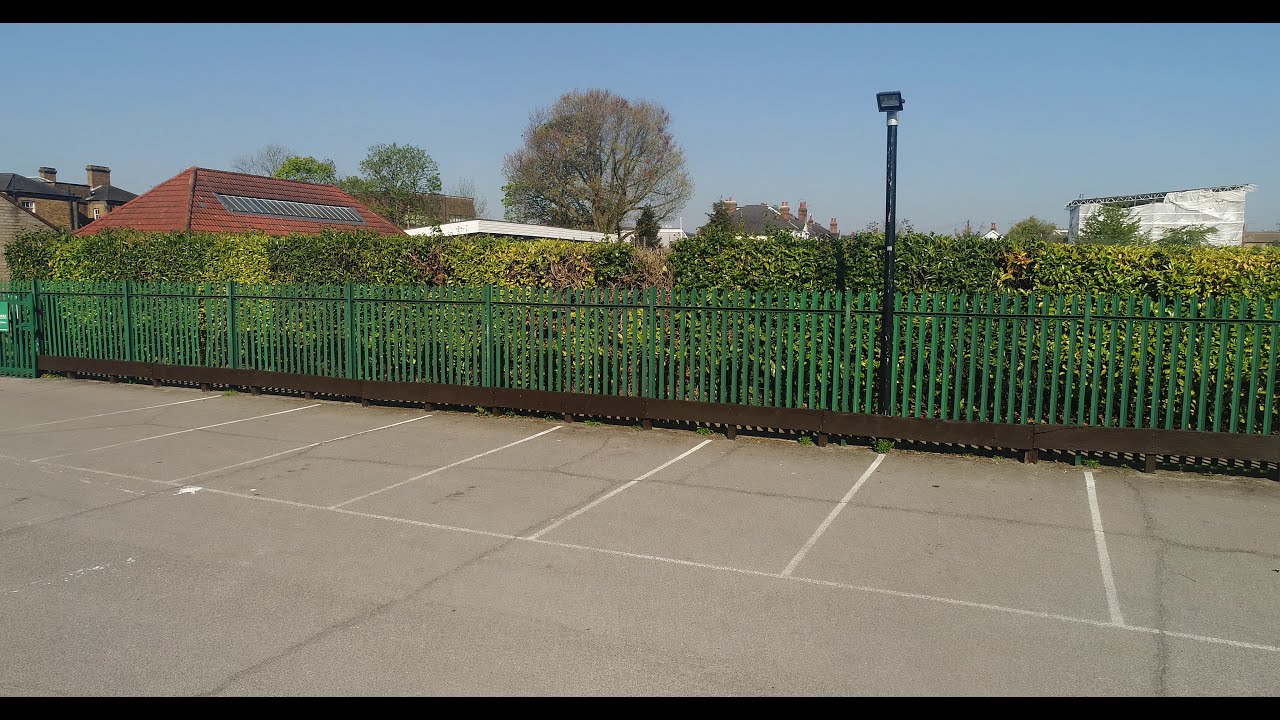The image presents a hyper-realistic outdoor scene of a parking lot with a gray asphalt surface meticulously divided by white lines delineating parking spaces. The area is bordered mid-frame by a green-painted picket fence, composed of vertical slats spaced apart, allowing glimpses of lush, dense shrubbery behind it. Breaking this greenery, a black lamppost ascends from the right side of the fence, crowned with a square lamp poised to illuminate the lot. Dominating the upper part of the photograph is a vibrant blue sky, completely unblemished by clouds. In this serene yet vivid setting, the background features elements suggestive of a suburban environment, including varied architectural structures: a prominent beige stucco building with two fireplaces to the left, a red-tiled roof suggesting a secondary building, and several white buildings of differing heights. The color palette is rich, with greens, blues, yellows, browns, blacks, grays, and whites harmoniously blending to enhance the realism of the scene. The image is devoid of human presence or any textual annotations, reinforcing its tranquil, almost pristine atmosphere.